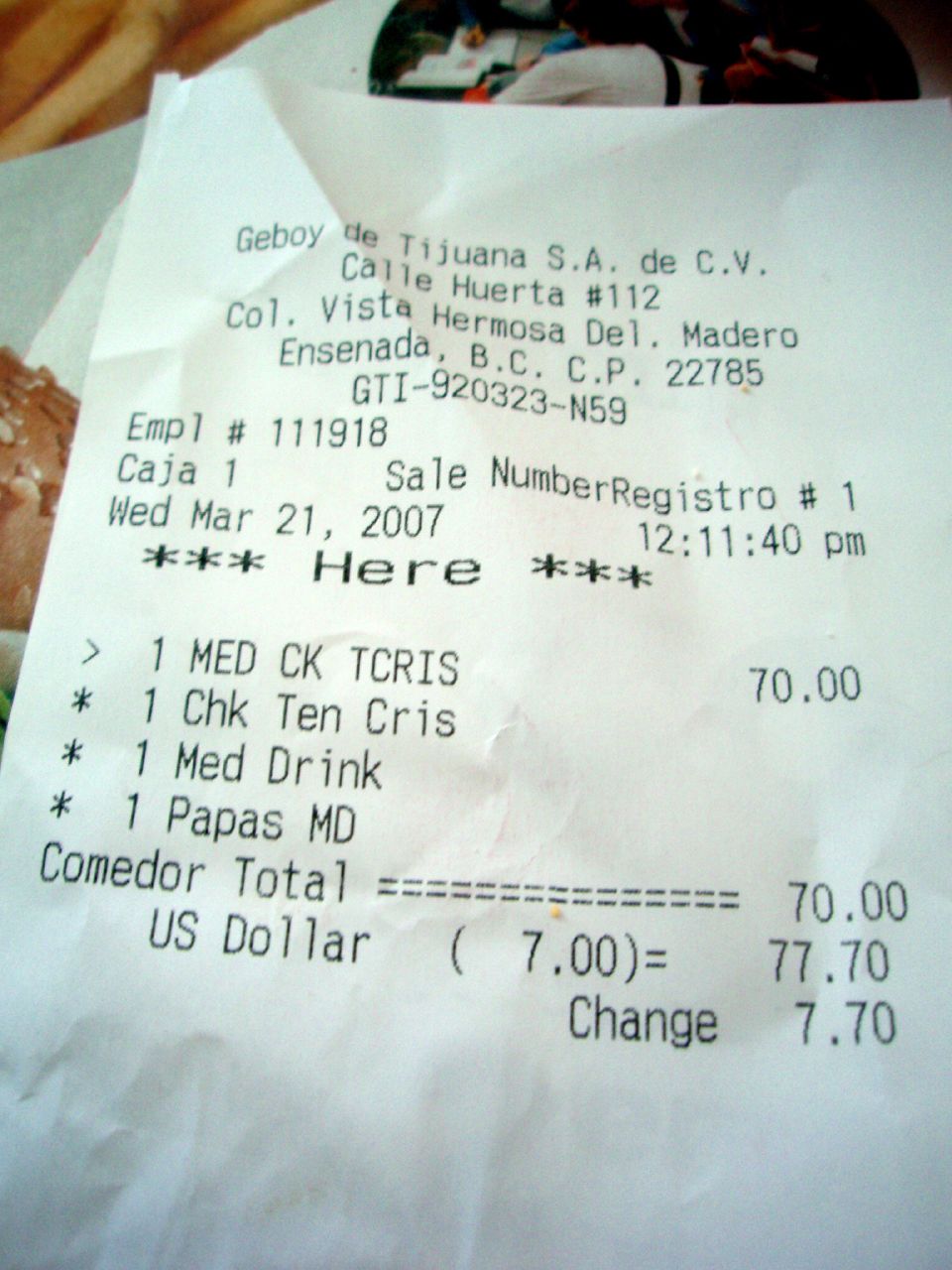An image shows a wrinkled, white paper receipt with black text, placed on a table. The receipt details a purchase from "Jeboi de Chioana S.A.D.C.V." located at "Calle Jareta 1112, Call de Vista Ramada de Madero, Ensenada, BC CP 22785." The transaction occurred on "Wednesday, March 21st, 2007 at 12:40 p.m." The receipt itemizes: "ONE MED CHICKEN TITRIS $70," "ONE CHICKEN TEND CRISP," "ONE MEDIUM DRINK," and "ONE PAPAS MD," totaling "$70," equivalent to "$7.70" in U.S. dollars, with the change also noted as "$7.70." Above the receipt, a photograph features a person with long black hair wearing a white shirt, along with some open books, fries, and hamburger buns in the surrounding area. The receipt itself has gray shadows towards the bottom, suggesting it is crumpled and placed on a cluttered surface.